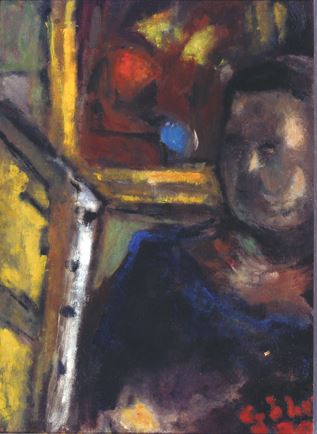This detailed descriptive caption would be:

The image depicts an impressionistic painting from the late 1800s or early 1900s, possibly rendered in watercolor or oil. Central to the artwork is a person, most likely a woman, dressed in a blue outfit. She stands or sits at the composition's center, facing away from the viewer, creating a sense of introspection. To her right, there is a painting within the painting, framed in gold or brown, possibly depicting flowers with hues of red, brown, and yellow. This additional painting adds depth to the scene and is slightly behind the main figure. On the left side, there is a structure that could be an easel, hinting that the central figure might be an artist, or it might be an open door with a brown wood frame and white highlights. The style leans toward impressionism, with minimal facial features, emphasizing eyes, a nose, and hair. The painting exudes a tranquil yet mysterious aura, inviting viewers to ponder the narrative and the emotions concealed within. A signature is visible in the lower right-hand corner, affirming the artist's identity.